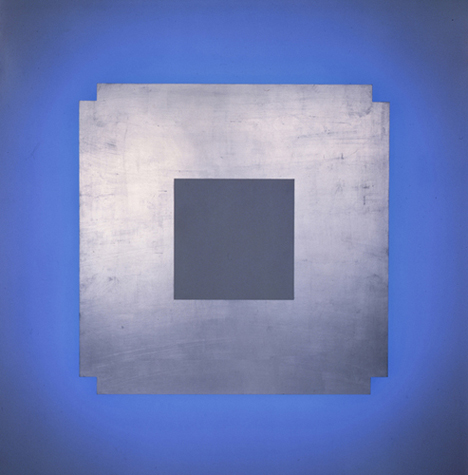This image is a square-shaped, abstract painting characterized by multiple layers and gradient effects. The backdrop features a blue square with its gradient edges darkening to almost a gray-black color at the corners, gradually lightening towards the center. In the middle of this backdrop lies a sheet of iron with a metallic, polished look, marred by small scratches and indents at the corners. Centrally positioned on the iron sheet is a regular gray square with no gradient, appearing flat and non-metallic. The setup gives a layered and texturally rich appearance, highlighted by a light source that emphasizes the upper sections of the metal plate, enhancing the metallic sheen. The overall composition, devoid of text or watermarks, is reminiscent of a minimalist, abstract art style.